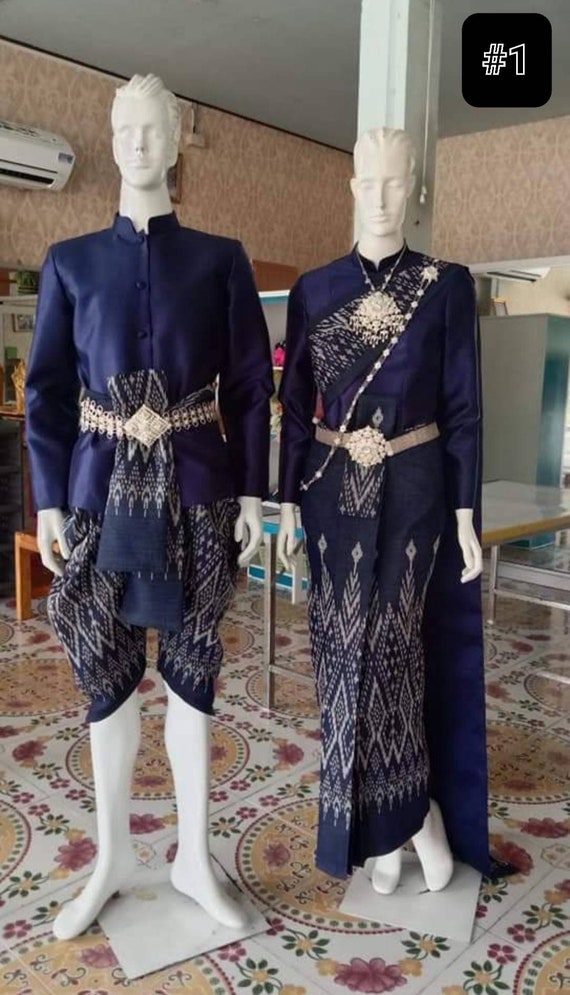In this detailed photograph, two mannequins, arguably representing a traditional wedding couple, are displayed in elaborate outfits that suggest cultural significance, possibly from India or Pakistan. The male mannequin dons a solid blue coat paired with matching blue shorts adorned with intricate diamond patterns. His ensemble is cinched at the waist with a belt made from the same material. The female mannequin wears a blue dress that extends to her ankles, featuring a skirt with a pattern matching the man's shorts, and a similar belt at her waist. She also sports an ornate white necklace. Standing indoors where ceramic tiles with mosaic designs cover the floor and floral print wallpaper in light brown and pink hues decorates the walls, the mannequins are framed by various interior elements. One stands in front of a white support column that runs from floor to ceiling, and in the background, a white air conditioning unit, tables, a chair leg, and a workspace are visible. An eye-catching black square with "#1" is found in the top right corner of the image.